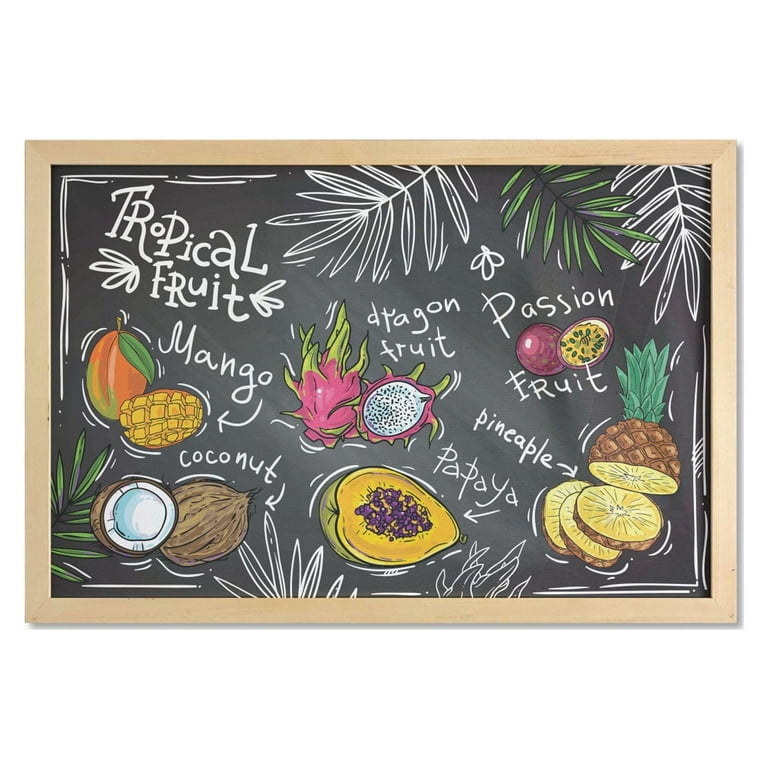The artwork is a horizontally rectangular piece, framed with a thin, light-grained wooden border and displaying a slight shadow along the bottom and right sides. The interior resembles a black chalkboard with a textured, dusty white wash in the center, enhancing the chalkboard effect. Positioned in the upper left corner, the inscription "Tropical Fruit" stands out in white. Surrounding this title, various colorful illustrations of tropical fruits—mango, dragon fruit, passion fruit, pineapple, papaya, and coconut—are artistically depicted and labeled with their names using white arrows pointing to each fruit. The fruits are carefully illustrated, some shown whole and others cut in half, featuring detailed colors such as red, yellow, green, orange, brown, and fuchsia. Accompanying the fruits, the top center extending to the top right displays a few artistically drawn leaves, with two in white and one in green. This intricate, visually engaging piece appears to capture the essence of a chalkboard drawing, blending vivid color illustrations with the simplicity of chalk-like white writing and sketches.